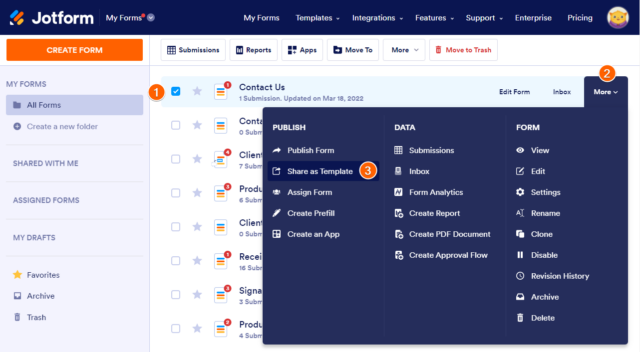The image displays the JotForm dashboard with various navigation and function elements vividly represented. In the upper left corner of the interface, the "My Forms" link is prominently displayed. Moving right along the top navigation bar, successive clickable links include "Templates," "Integrations," "Features," and "Support," each accompanied by a pull-down menu. Following these is the "Enterprise Pricing" link. At the far right, there's a circular icon featuring an orange cartoon creature.

Beneath this top bar, a vibrant orange "Create Forms" button with white text is positioned to the left. To its right, functions like "Submissions," "Reports," "Apps," "Move to More" with a pull-down menu, and "Move to Trash" - highlighted in red while the others are in black font - are aligned.

On the far left side of the interface, a vertical navigation strip lists options such as "My Forms," "All Forms," "Create a New Form," "Shared with Me," "Assigned Forms," "My Drafts," "Favorites," "Archive," and "Trash." The user's current selection is "All Forms," distinguished by a darker, purple-gray background compared to the lighter purple-gray background of the other options.

In the main content area, the visible entry is labeled "Contact Us." A partially obscured list of other forms follows this entry. A blue pop-up notification appears in the center of the screen, showing various numerical badges: a '1' next to "All Forms" within an orange circle, a '2' indicating "More" with a drop-down, and a '3' indicating "Share as Template."